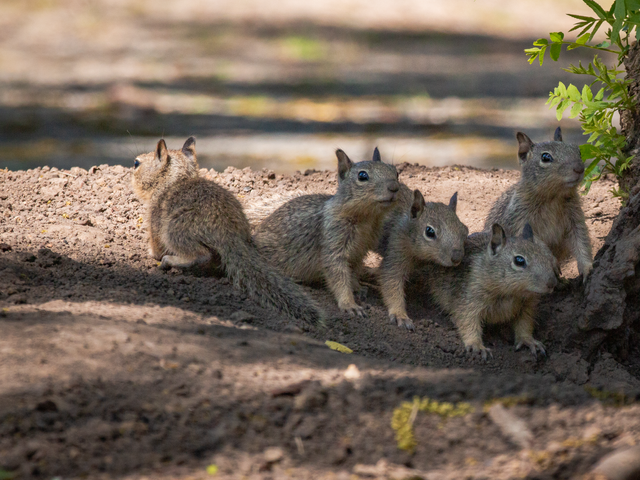The photograph captures a group of five squirrels against a backdrop of rocky, recently disturbed soil. Four squirrels are positioned to the right, their bodies turned slightly to the right while facing towards the camera, but their gaze is directed towards something off-screen to the right. The fifth squirrel, positioned to the left of the group, has its back turned to the camera, offering a clear view of its long, bushy tail. All the squirrels share the same fur coloration, a mix of brown with some hints of gray and tan. They all have black eyes that hint at their alert curiosity. To the right edge of the image, a partially out-of-focus tree or bush with green leaves can be seen, adding a touch of greenery to the earthy surroundings. The background remains blurred, providing little detail about the exact location but giving a sense of an outdoor, natural habitat.